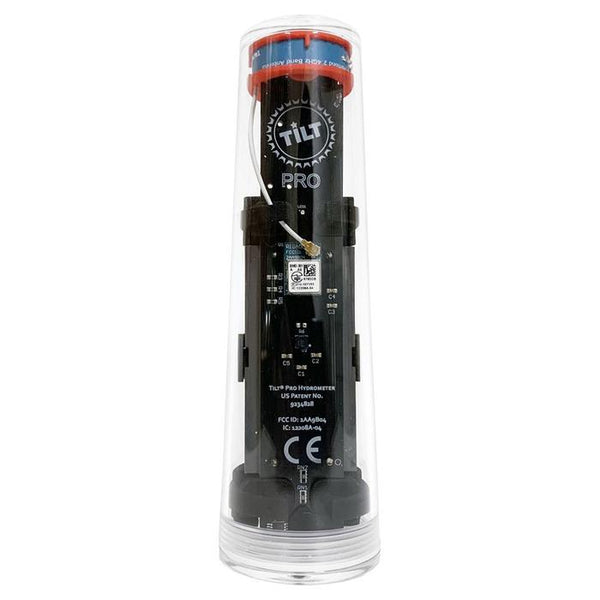The product photograph depicts an electrical meter, encased in a clear acrylic plastic cylinder, giving it a distinct appearance of floating in an empty, white, featureless void. This aesthetic is commonly used in commercial settings such as online shops, listings, catalogs, or websites to highlight the product. The black rectangular meter is positioned vertically in the clear cylindrical container, which has a curved rounded top featuring blue and red trim. White text is displayed prominently on the device; at the top, within a circle, it reads "TILT," followed by "PRO" underneath. Additional text, including "hydrometer," a U.S. patent number, and "CE" are inscribed further down on the meter, although some smaller details are difficult to discern. The image is rectangular, with the horizontal sides being twice the length of the vertical sides, creating a balanced yet striking display of the product within its clear casing.